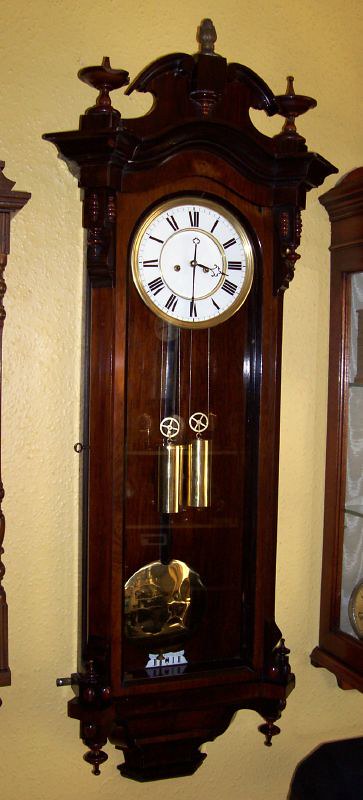An antique wooden wall clock, displaying masterful craftsmanship with intricate finials and ornate carvings at the top, stands prominently against a textured yellow wall. The clock, approximately the length of a grandmother clock, features a polished brown finish and exhibits a timeless elegance. Its white clock face is encircled by a gold bezel, housing Roman numerals and detailed minute and hour hands, though it notably lacks a second hand. A pair of hanging weights and a pendulum are visible within the clock's elongated body. Flanking the central clock are glimpses of two similar timepieces, adding to the vintage ambience of the setting.